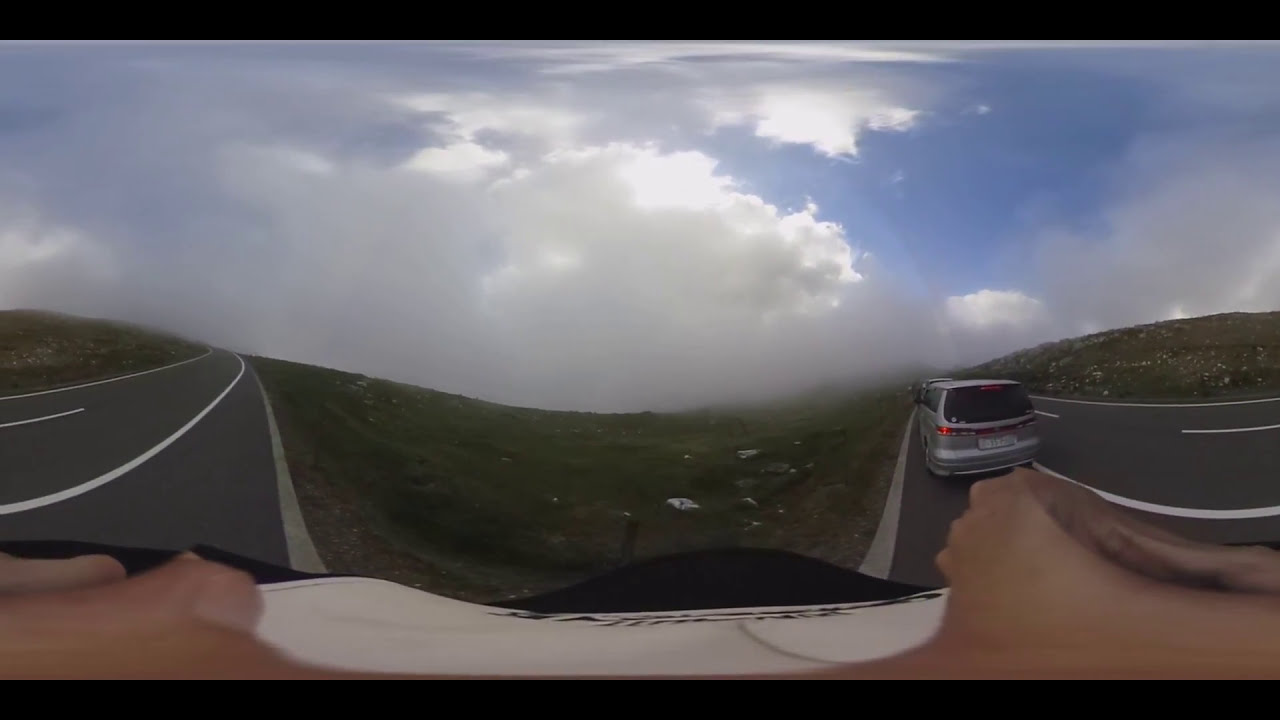In this surreal, edited image, two winding roads stretch across a hilly, verdant landscape under a vibrant blue sky mottled with gray and white puffy clouds. The picture is framed with thin horizontal black stripes at the top and bottom, enhancing its otherworldly charm. On the smooth, dark gray concrete of each road, freshly painted white lines delineate lanes, with the right road featuring a silver van driving away. The left road remains empty, emphasizing the van's solitary movement.

At the center, the roads slope inward towards a lush, green grassy embankment, peppered with a few white stones. The grass continues outward, creating a tranquil, pastoral setting amid the curving roads. A pair of hands, stretched out from the bottom corners of the image, appearing to hold or frame it with a white cloth, adds a peculiar, almost cinematic perspective, possibly hinting at the image being a highly distorted or panoramic view. The entire scene exudes an elevated, mountainous atmosphere, with clouds seemingly brushing against the hills, evoking a sense of being high above sea level.